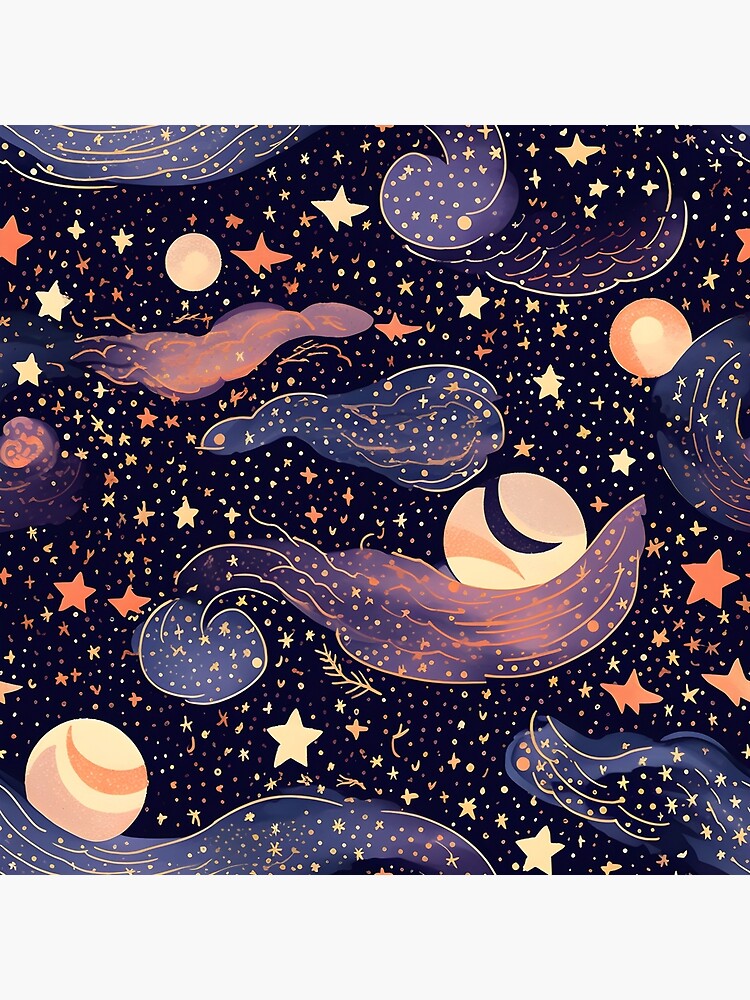The artwork is a vertical rectangular piece that depicts a night sky scenario. The background is predominantly black, teeming with thousands of stars in hues of yellow, orange, and white. Interspersed among the stars are several planets, rendered in orange and yellow, with one distinctive planet featuring a smile cut out of it. The sky also contains various cloud-like formations that are outlined in different shapes, including paisley and amoeba-like figures, through which the dark sky can be seen. Swirling bands of purple, blue, and white add a dynamic texture to the scene, creating the impression of a celestial dance. Despite the crowded star field, the artwork retains a sense of whimsy with its stylized clouds and vivid planetary bodies, offering a unique interpretation of an imagined outer space.